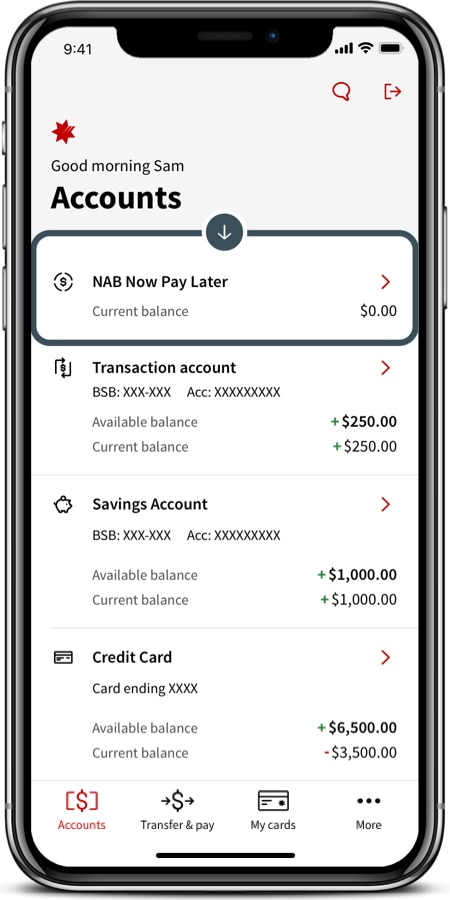This image depicts a smartphone screen showcasing a financial application interface. At the top left corner, the time is displayed as 9:41, while the top right corner features three icons: a Wi-Fi signal, cellular signal, and battery level indicator.

Beneath the status bar, text reads "Good Morning Sam Accounts," followed directly below by a downward-facing white arrow. The screen is divided into four sections, each containing specific account information.

- The first section lists "NAB, Now Pay Later.”
- The second section details "Current Balance," which shows $0.00 on the right side.
- The third section provides information on a "Transaction Account" with the format "BSB: XXX-XXX" and "ACC: XXXXXXXXXX," followed by an available balance of +$250.00 and a current balance also of +$250.00.
- The fourth section begins to show details of a "Savings Account," referenced again with "BSB."

Overall, this account summary on the financial app gives a clear breakdown of the user's available funds and current balance across different sections.